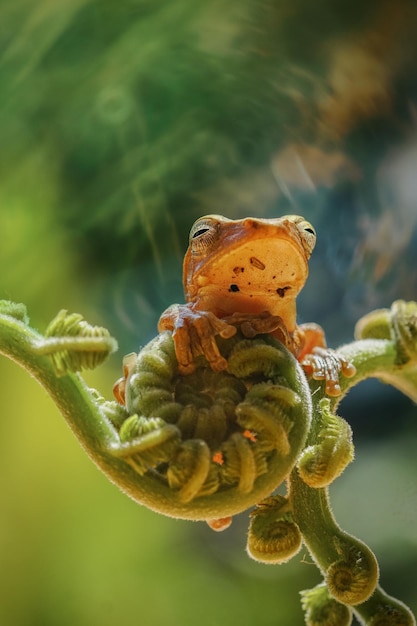This image captures an orange-yellowish tree frog with little suction cups on its toes, seemingly suspended on a vibrant green, spiraled vine or plant. The frog is positioned frontally and slightly upwards, exhibiting its two front legs clinging to the plant on the left side while its back leg is anchored on another vine emerging from the right. Its striking eyes feature black slits against white surrounds, lending it a unique and engaging gaze. The background, a blend of blurred greens with hints of white and brown hues, ensures the focus remains solely on the vividly colored amphibian and its intricate perch. The curled vines, perhaps symbolizing new growth, add a touch of complexity and natural beauty to the scene.